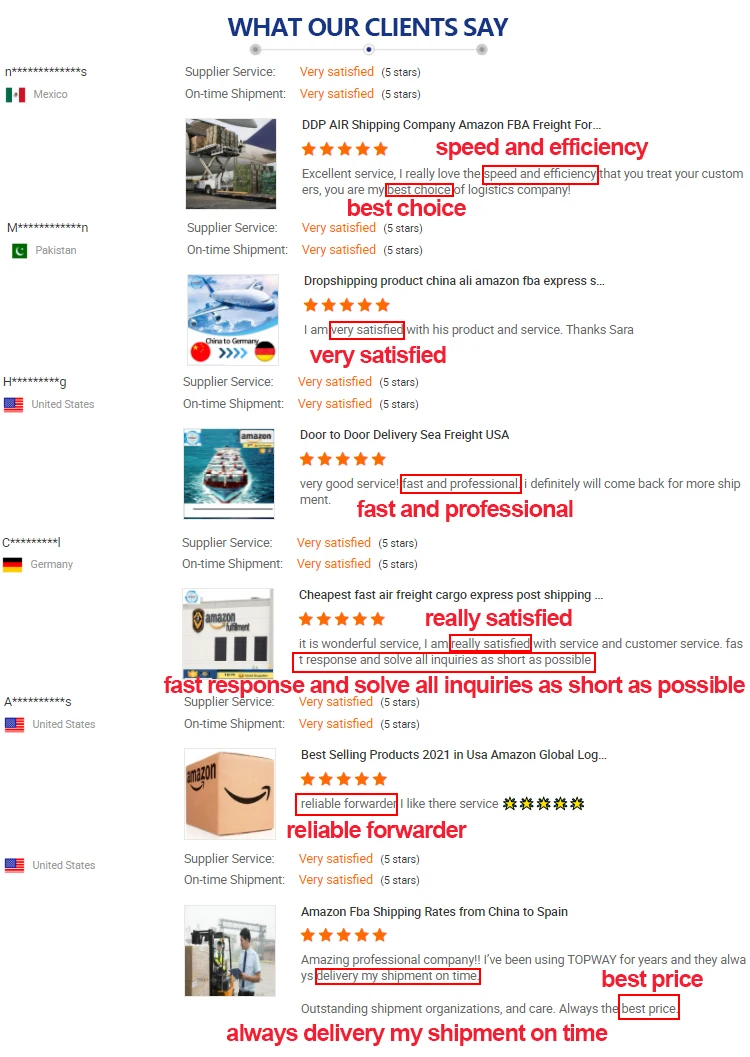The screenshot displays a detailed web page result showcasing client testimonials and ratings for shipping services across various countries. At the top, headings highlight aspects such as "Supplier Service" and "On-Time Shipment." 

For Mexico, a photograph captures the efficient loading of cargo into a freight aircraft, accompanied by descriptors like "speed," "efficiency," and a "five-star" rating. 

Pakistan's section features an image of a cargo plane in-flight, with keywords such as "drop shipping product," "China," "Amazon FBA Express," "door-to-door delivery," and "sea freight."

The United States section is filled with comments praising "fast and professional" services, most of which are rated five stars. A particular note is made of Amazon FBA shipping rates from China to Spain, and the overall theme is one of high satisfaction.

Germany's testimonials mention "fast response" and efficient problem-solving, labeling the service as a "reliable forwarder." 

Throughout the listing, the dominant impression is consistent five-star ratings, highlighting client satisfaction with timely deliveries and best-choice shipping options across all mentioned countries, including frequent mentions of the United States and Germany.

Absent is an overarching heading for the company providing these services, but it's evident that the testimonials focus on a range of shipping methods, including drop shipping, DDP air shipping, and Amazon-related logistics. The repeated five-star ratings emphasize reliable and satisfactory client experiences.